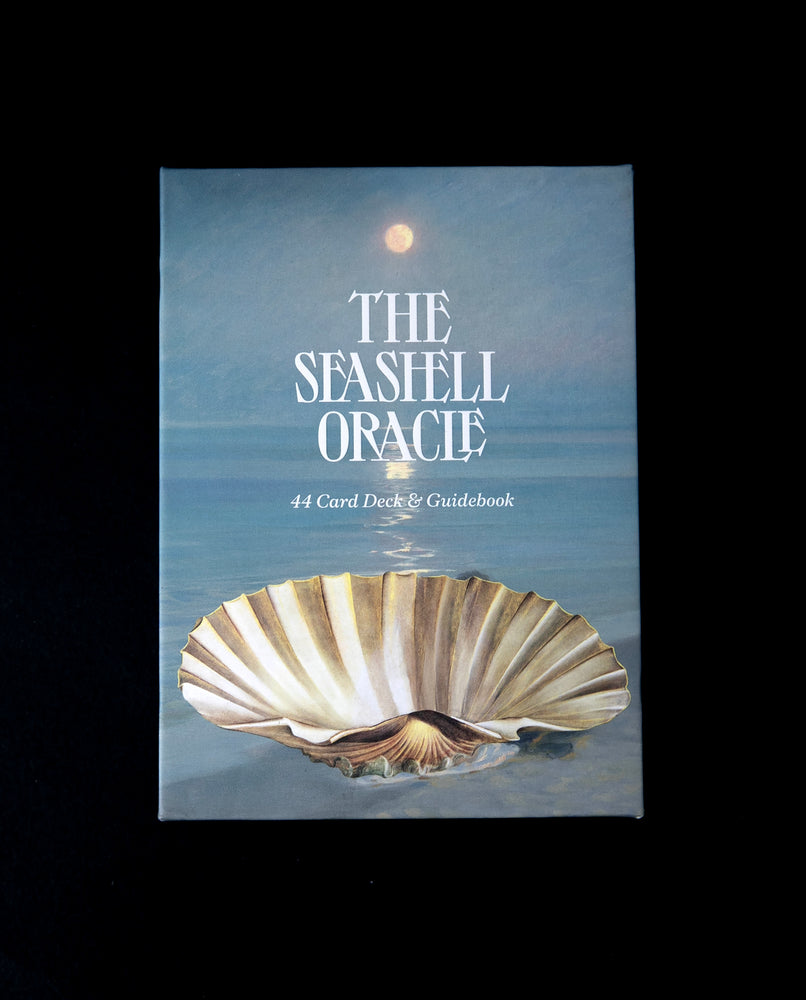This image features a book cover with a distinctive black border, presenting a vertical, rectangular composition. The centerpiece is a beautifully illustrated scene with a blue backdrop that resembles a painted artwork. In bold, all-capital letters, the title "THE SEASHELL ORACLE" is prominently displayed in a unique font, followed by the description "44 CARD DECK AND GUIDEBOOK" also in white lettering. Below the text is a large, visually striking seashell, characterized by a rich brown and white coloration. The seashell rests on what appears to be a beach, with the expansive sea extending into the background. Above, a celestial body—interpreted as either the sun or the moon—casts radiant light, which reflects off the shimmering water below, adding a serene and mystical quality to the scene.